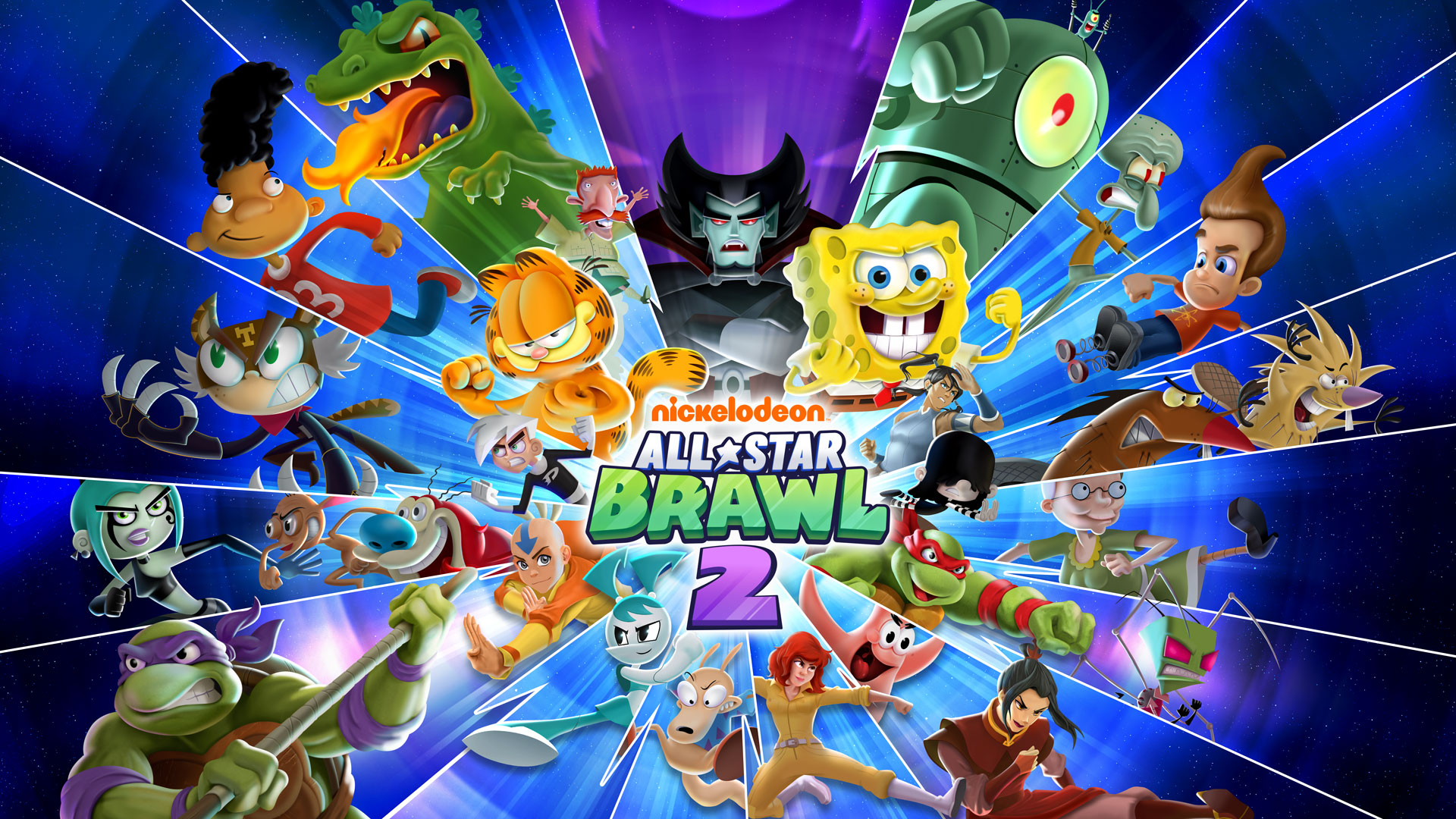This vibrant digital render advertises Nickelodeon's game, All-Star Brawl 2, with an electric blue and galaxy-like background that fades into purples and blacks at the edges. At the heart of the image, bold text spells out "Nickelodeon" in orange, "All-Star" in white with a star symbol, "Brawl" in green, and a prominent "2" in purple. Surrounding this central text, a dynamic array of Nickelodeon characters shoot outwards as if in a cascading spiral, separated by white lines. Featured prominently are beloved characters like SpongeBob SquarePants positioned above the Nickelodeon text to the right, Garfield to the left, and a Dracula character at the very center. Also included are icons such as Plankton, Squidward, Jimmy Neutron, the Angry Beavers, the Teenage Mutant Ninja Turtles, Patrick Star, and Rocko from Rocko's Modern Life. All characters and elements combine to create an energetic, high-quality image that encapsulates the spirited and competitive atmosphere of the game.